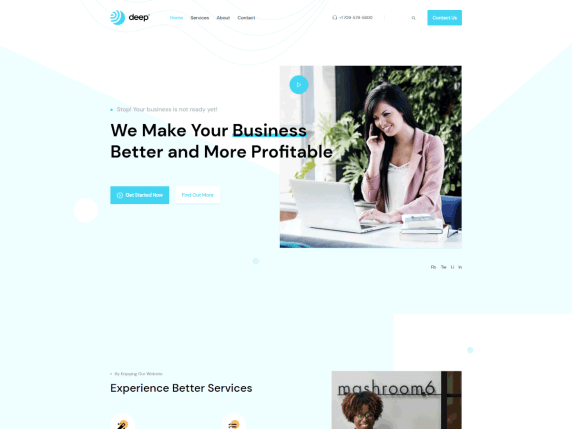The image showcases an advertisement with a clean, white background. In the upper left corner, the word "Deep" is prominently displayed next to a bright blue logo featuring a circular design with white, spiraling lines. Dominating the central part of the advertisement, bold text proclaims, "We Make Your Business Better and More Profitable." Just beneath this text is a large, prominent square image depicting a woman multitasking; she is seated at a computer, holding a cell phone in her right hand while typing on a laptop with her left hand.

Below this main section, a partially cut-off advertisement catches the eye. The text reads, "Experience Better Services," accompanied by another cut-off image that seems to introduce "Mashroom 6." This ad features a black woman with short hair and glasses, although the image is only partially visible.

Across the very top of the overall image, a header line provides navigation options, indicating links to various sections of a website. The dominating color scheme outside of the ad content utilizes black and blue text against a pristine white background, offering a clean and professional look.